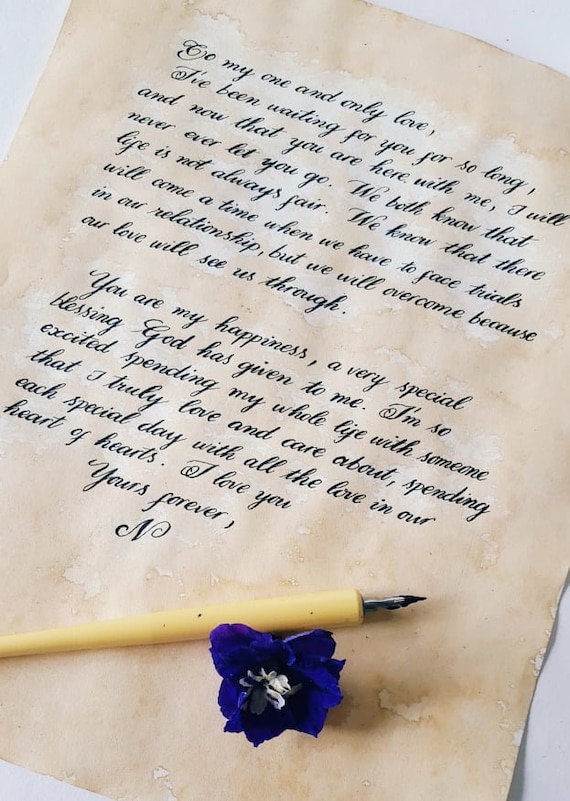The image depicts an aged, cream-colored piece of calligraphic paper adorned with a handwritten love letter in elegant cursive script. The letter begins with the heartfelt words, "To my one and only love," and continues to express deep emotions and unwavering commitment: "I've been waiting for you for so long and now that you are here with me, I will never ever let you go. We both know that life is not always fair. We know that there will come a time when we have to face trials in our relationship, but we will overcome because our love will see us through. You are my happiness, a very special blessing God has given to me. I am so excited spending my whole life with someone that I truly love and care about. Spending each special day with all the love in our hearts of hearts. I love you, yours forever." The letter is signed with the initial "N" and is accompanied by a vintage calligraphic pen with a tan wooden handle and a metal tip. Beside the pen lies a small, vivid purplish-blue lavender flower, adding a touch of color and sentiment to the scene. The entire paper appears weathered, as though it has been lovingly preserved over time, with its artificial aging and water-worn marks evocative of enduring love.